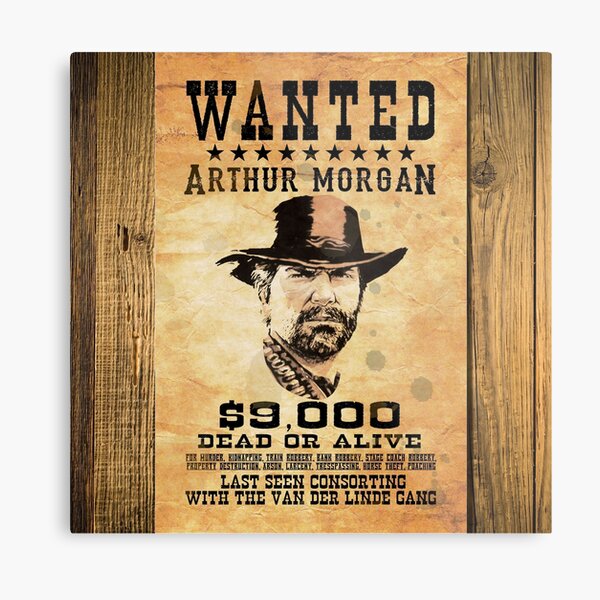This photo captures a classic Wanted poster mounted on a vertical, light brown wood plank background. The poster itself is a tea-stained, light brown piece of paper with distressed edges, giving it an authentic, aged appearance. Centered on the poster, in a western font, are the bold words "WANTED" at the very top, flanked by a line of nine dark brown stars below it. Right underneath, in a slightly lighter brown font, the name "Arthur Morgan" is prominently displayed. 

Following the name, there's a detailed drawing of Arthur Morgan, showcasing a rugged-looking man donned in a wide-brimmed cowboy hat. His stubbly beard and intense, mean expression add to his outlaw persona. Around his neck, there appears to be a strap, possibly resembling a bullet belt. Below his picture, the bounty of "$9,000" is printed in large, dark brown numbers, accompanied by the ultimatum "DEAD OR ALIVE". 

Further down, although the text is less clear, it lists several offenses such as larceny, arson, trespassing, horse theft, and stagecoach robbery. The last line reads, "Last seen consorting with the Van Der Linde gang." The entire poster is framed with a light gray border, adding a finishing touch to this evocative piece of western themed art.